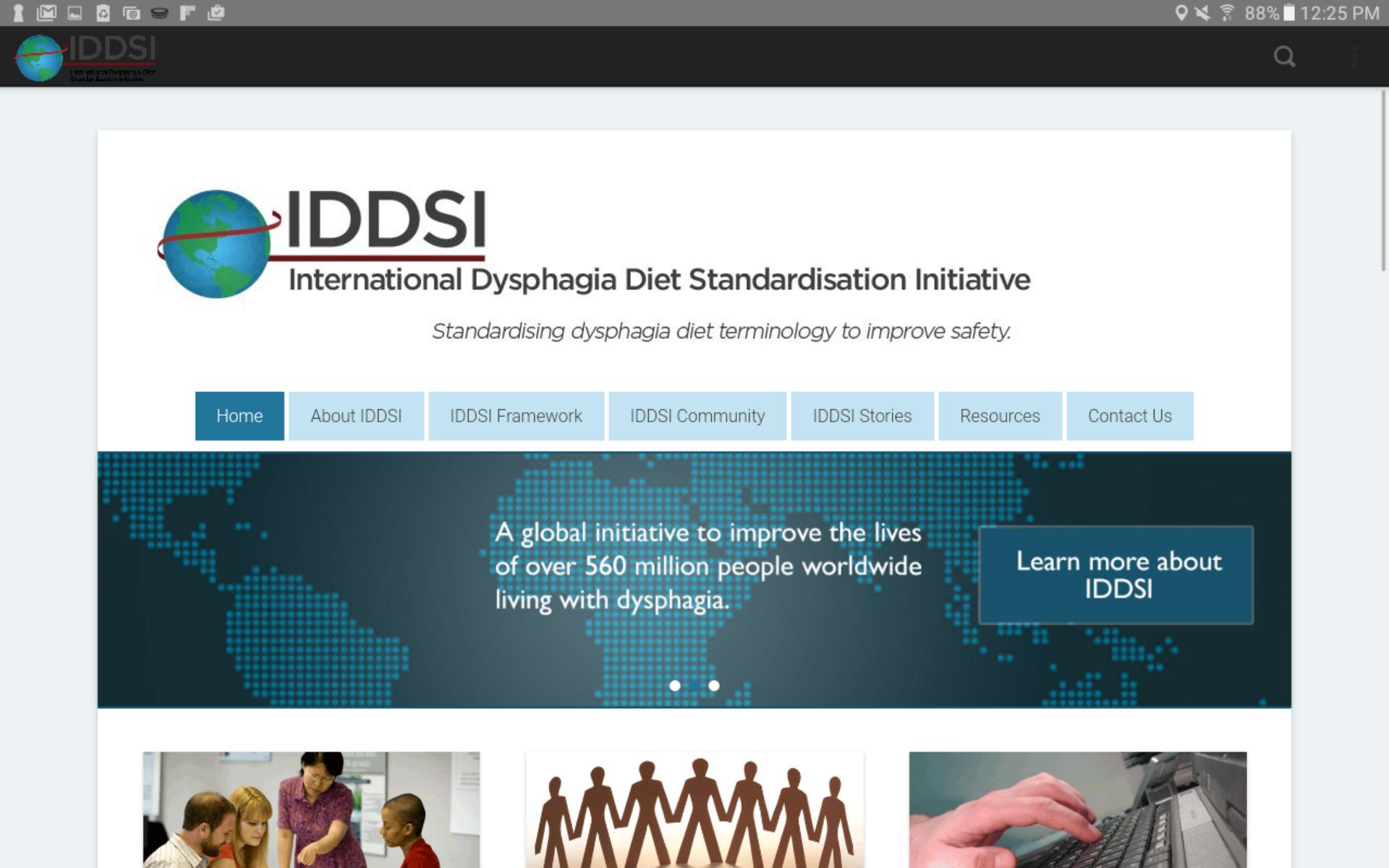This screenshot highlights the International Dysphagia Diet Standardization Initiative (IDDSI) webpage. The topmost section of the image features a gray bar containing various computer symbols such as a keyhole icon, Gmail, Photos, Headphones, Text Message, an unidentified icon, a large 'F', a checkmark, and indicators for location, Wi-Fi signal (at 88%), battery status, and the current time of 12:25 PM. 

Beneath that, a black bar displays a globe with a red swirl, accompanied by the underlined acronym "IDDSI" in red. Although something else is written in red text under the acronym, it is illegible. To the right in this black bar is a magnifying glass icon. The webpage background is gray, framing a central white block. This block features the globe again, with the red ribbon looping behind it and underlining "IDDSI." Below this underline, the full name, International Dysphagia Diet Standardization Initiative, is written with a centered tagline: "Standardizing Dysphagia Diet Terminology to Improve Safety."

Further down, there are several blue boxes offering navigation choices: Home, About IDDSI, IDDSI Framework, IDDSI Community, IDDSI Stories, Resources, and Contact Us.

The subsequent section features a dark image showing a pixelated world map, highlighting parts of North America, South America, Europe, Asia, Africa, and Australia. Overlaid in white text is the phrase, "A Global Initiative to Improve the Lives of Over 560 Million People Worldwide Living with Dysphagia." To the right, a blue box with white text reads, "Learn More About IDDSI." Two white dots at the bottom of the map suggest the presence of additional images accessible by navigating the dots.

The final segment of the screenshot, partially cut off, presents three images. The first image shows a group of four people: a man with a beard and a balding spot wearing a white shirt, a red-haired woman in a red shirt, an Asian woman in a purple shirt pointing at something on a desk, and a bald person of indeterminate gender in a red shirt. Behind them are some unreadable signs positioned on the wall. The second image depicts seven stick figures holding hands in a curved formation. The third image shows a left hand poised above a keyboard, with the index finger resting near the 'D' key and the other fingers idle.